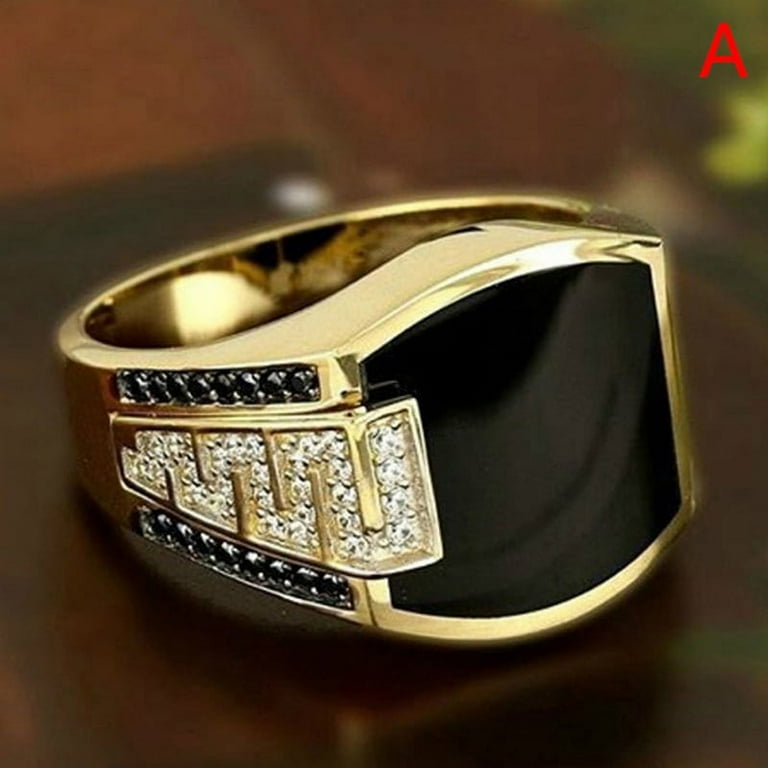This detailed image showcases a close-up of a gold ring, tilted to display its intricate design. The ring's face features a large, matte black, square-shaped stone, likely black onyx. Overlaying the stone is a striking zigzag encrusted with sparkling diamonds, resembling a snake. Flanking this are rows of black diamonds or black stones, possibly black onyx, adding to its elaborate design. The background of the image is artistically blurred with shades of brown and green, drawing full attention to the ring. In the upper right-hand corner, there is a small, red capital letter "A". The composition and details suggest this ring, perhaps a signet style, is large and masculine-looking, making it a statement piece.